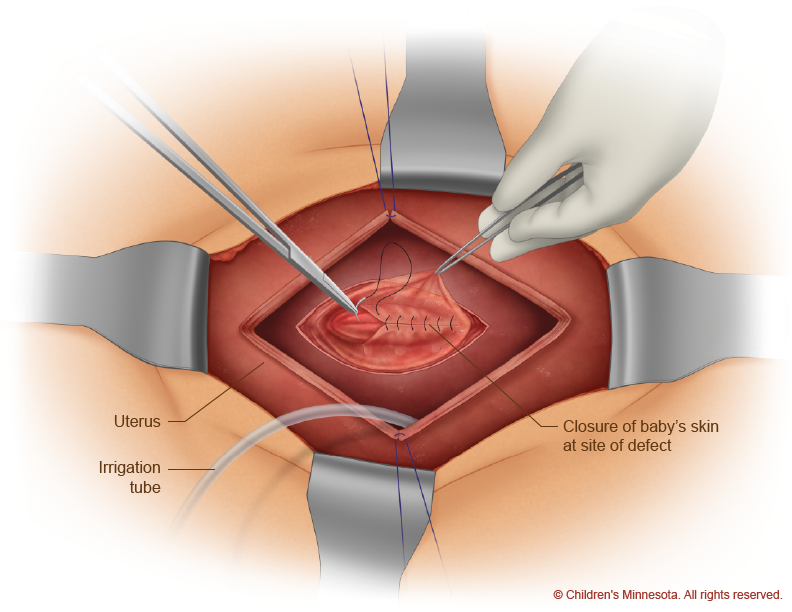The image is a detailed digital illustration of a surgical procedure, highlighting the closure of a baby's skin at the site of a defect. The artwork, copyrighted by Children's Minnesota, features different elements in a clear and color-coded manner. At the bottom right, the illustration notes the copyright in red text against a white background. The primary focus is on a peachy-pink outer layer, representing the skin, which is being held open by four gray clamps. 

Beneath the skin, a reddish-pink area, labeled as the uterus, is exposed. An irrigation tube is inserted into this area, emphasizing the procedural aspect of keeping the surgical site clean. In the center, a pair of hands, possibly gloved, are working meticulously. One hand, descending from the top, holds tweezers while another tool resembling scissors holds a thin needle and thread, actively stitching the skin. Arrows and labels provide additional context, with prominent text indicating "closure of baby's skin at site of defect." The detailed representation captures the complexity and precision required in such medical procedures.